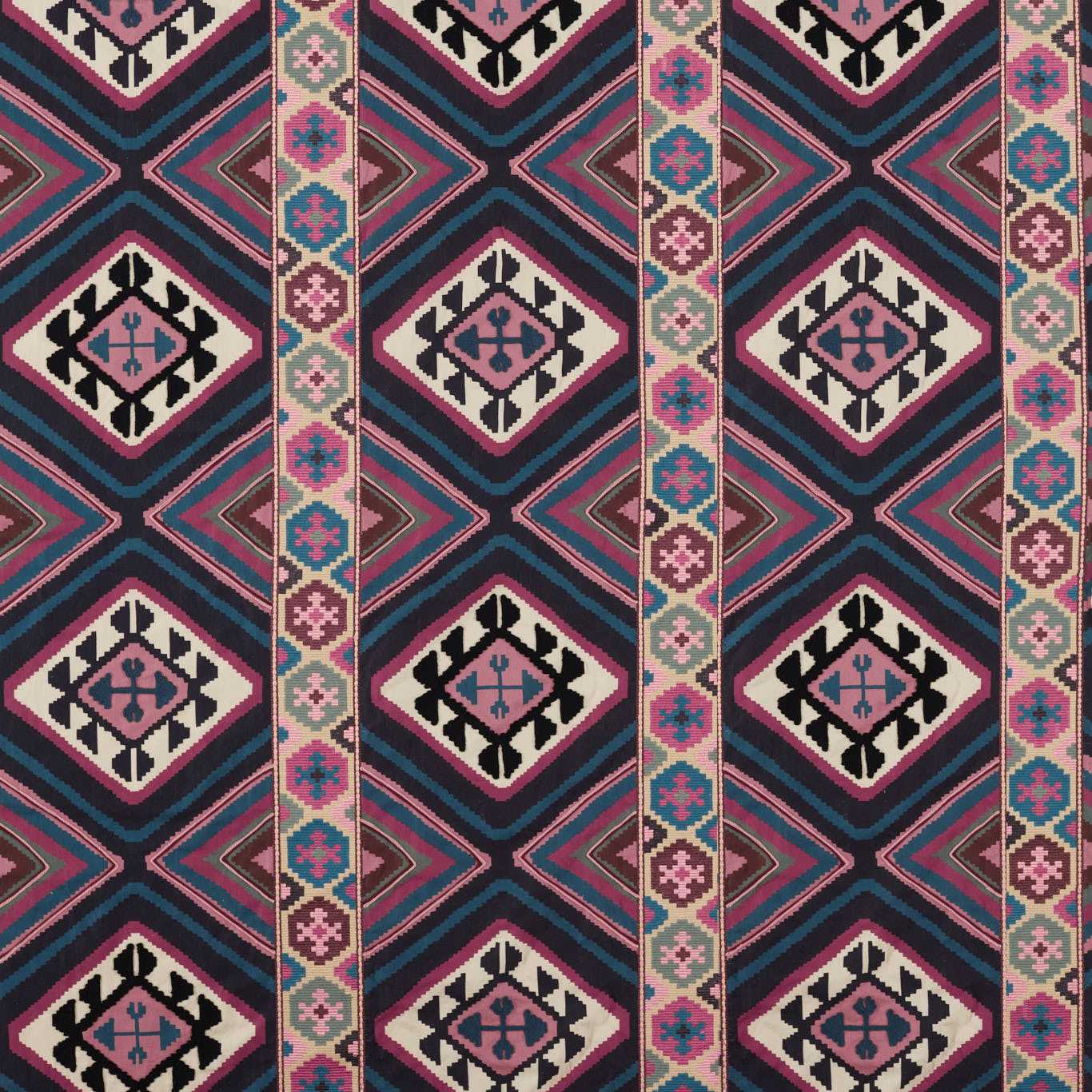The image depicts a hand-woven fabric or carpet with a vibrant, intricate Aztec-inspired design, viewed from a top-down perspective. The overall pattern is a series of alternating wide and narrow vertical stripes. The wider stripes feature diamond shapes with black backgrounds encircled by thin blue and pink lines, and inside is a white area with complex Aztec motifs, resembling a wrench and a two-sided arrow in shades of black, pink, and blue. The narrower stripes consist of hexagonal, snowflake-like designs alternating in a sequence of colors: green, pink, blue, burgundy, with pale pink centers. Dominated by deep pink (fuchsia) and black, the fabric also incorporates hues of blue, dusty rose, beige, white, and maroon, creating a repetitive yet vibrant geometric pattern characteristic of traditional Native American craftsmanship.